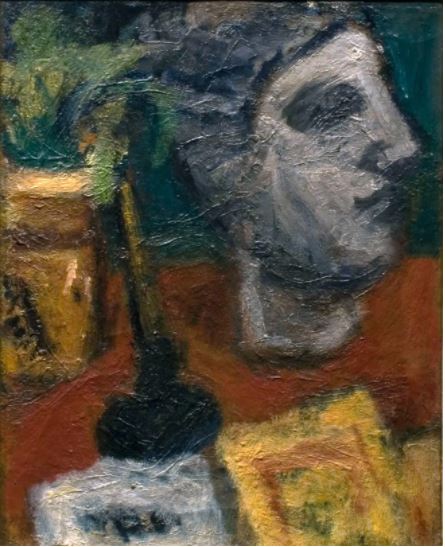The image is an abstract painting on a textured canvas that appears almost stone-like. Dominating the scene is a grey bust of a human figure with prominent dark eyes and slicked-back hair, looking to the right. The figure, possibly a man, wears a red top, and a somewhat indistinct paper or patch is visible on his shirt. In front of him, resting on a surface that could be a desk or table, are two wobbly-edged blocks—one yellow and one white with black markings. To his left stands a plunger-like object and behind him, adding to the composition’s surreal quality, is a square vase housing green leaves. A black candlestick holder with a candle also shares space near the bust. The overall scene is blurred, contributing to its abstract nature and making it challenging to discern the exact subject, but it evokes a mix of mundane and fantastical elements.